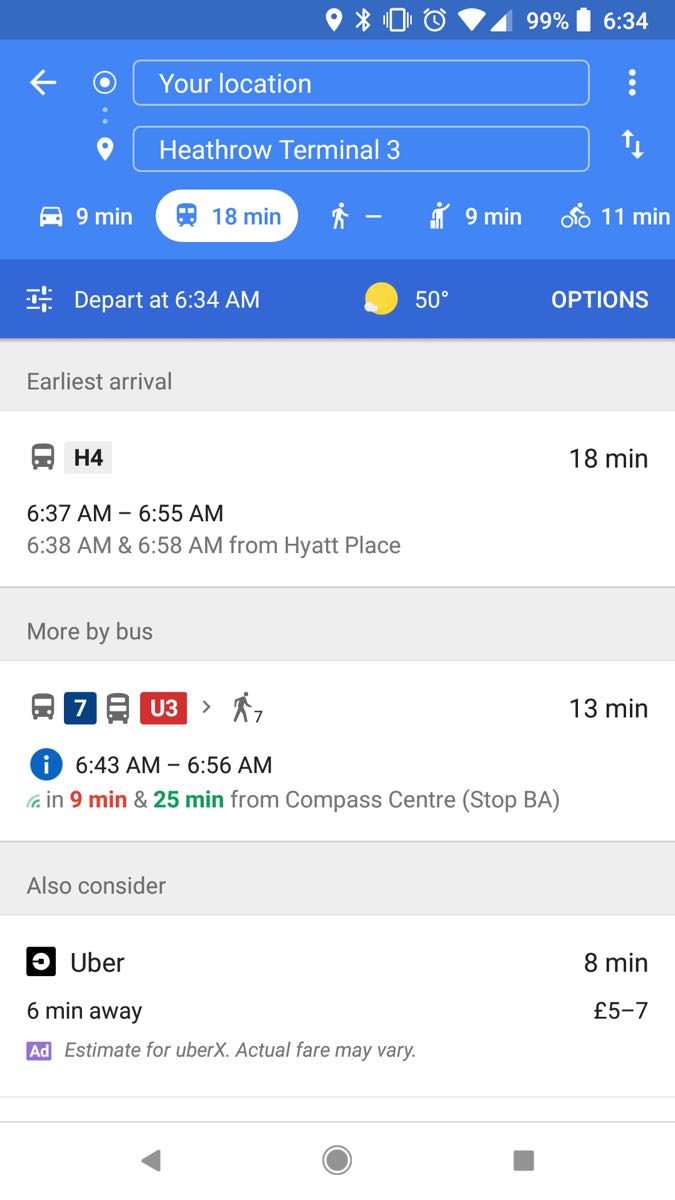A person is exploring various ways to reach Heathrow Terminal from their current location. The digital display indicates departure at 6:34 AM and provides three main options:

1. **Bus H4**:
   - **From Hyatt Place**:
     - Departure: 6:37 AM
     - Arrival: 6:55 AM
     - Duration: 18 minutes
   - **From another nearby stop**:
     - Departure: 6:38 AM
     - Arrival: 6:58 AM
     - Duration: 20 minutes

2. **Bus U3**:
   - **From Compass Centre, Stop BA**:
     - Departure: In 9 minutes
     - Duration: 13 minutes

3. **Number 7 Blue**:
   - Departure: In 25 minutes.

Additionally, the display provides Uber as an option:
   - **Departure**: 6 minutes away
   - **Duration**: 8 minutes
   - **Cost**: £5-£7 (Estimate for UberX; actual fare may vary). 

The travel information is neatly organized to help the user choose the quickest or most convenient route to their destination.